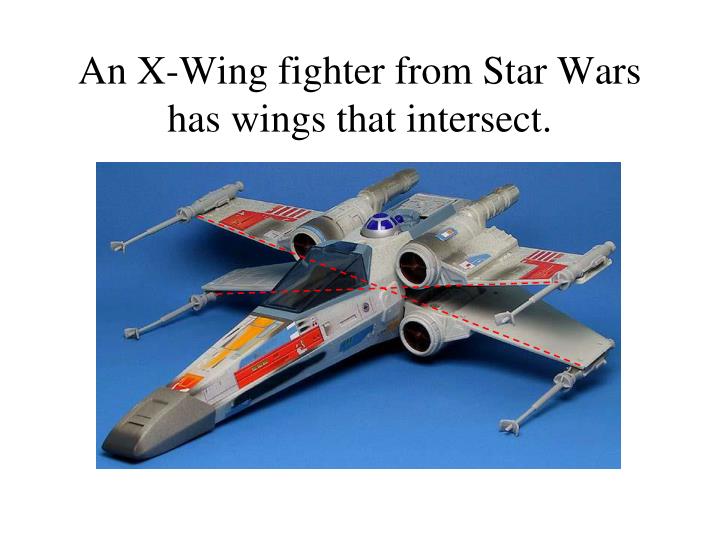The image depicts a detailed and vibrant poster of an X-Wing fighter from Star Wars. Set against a solid blue rectangular background, the X-Wing is shown at an angle, with the back end positioned in the upper right corner and the front end pointing towards the lower left. The plane is predominantly light gray, with a dark gray cap at the very tip of its nose. Distinctive red lines accentuate the four wings, which intersect each other, a hallmark design feature of the X-Wing. At the ends of these wings, there are missile-like guns, one on each side, akin to those found on military aircraft. Three engines are visible: two on the right and one on the top left, suggesting a fourth out of view. Near the cockpit, the small, recognizable dome of R2-D2 can be seen, marked by blue sections and a blue circle on top. Large black text at the top of the poster reads, "An X-wing fighter from Star Wars has wings that intersect," providing context to the iconic spacecraft.